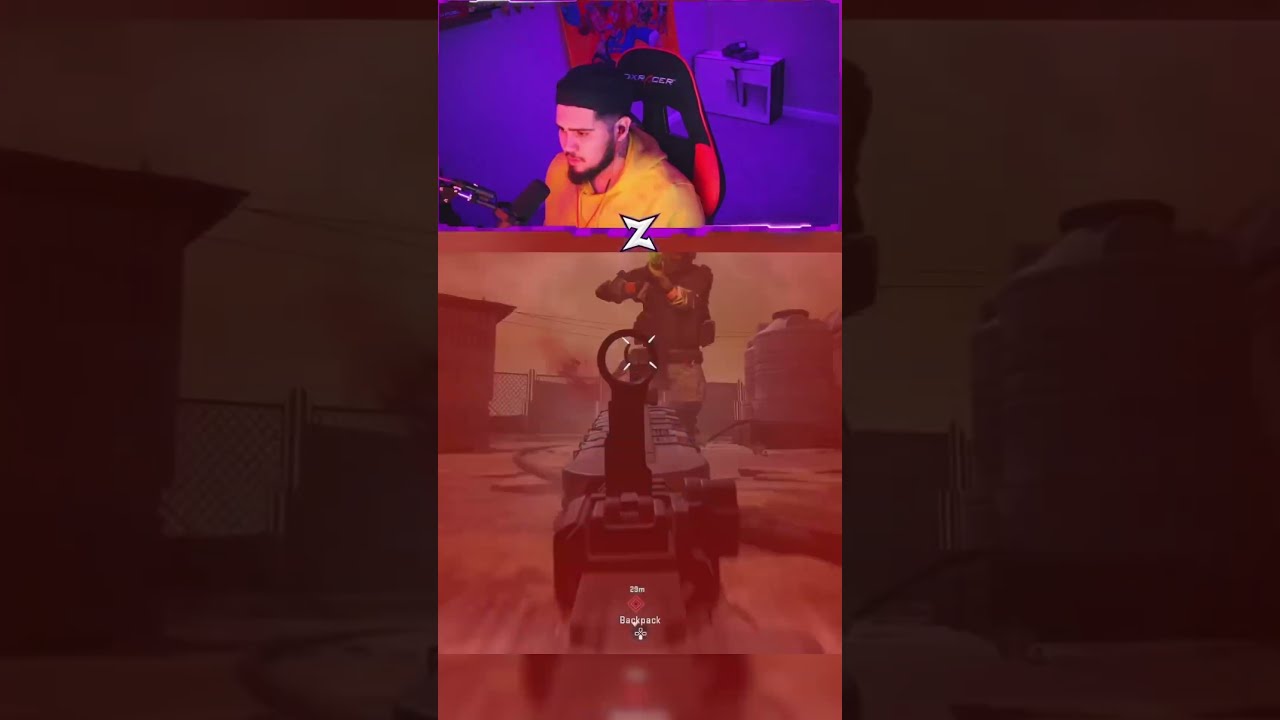In a detailed image, we see a streamer playing a first-person shooter game. He sits in a black-and-red DXRacer gaming chair, within a black-and-red tent. The streamer, who has lighter skin, dark hair, a black beard, and mustache, wears a backward baseball cap and a yellow hoodie. He's talking into a silver mic stand with a black microphone positioned to his right. Behind him, the wall glows blue, adorned with a red-and-blue poster. The image is a tall rectangle, with the top portion showing the streamer in his setup, and the bottom part displaying the game he is playing. The game screen features a red-tinted scene, indicating the streamer has just been shot. The viewpoint shows a weapon with a metal post and a round sight, aimed at an enemy hovering above the downed player. The borders of the image are an enlarged, slightly grayed-out version of the main image, providing a distinct frame.